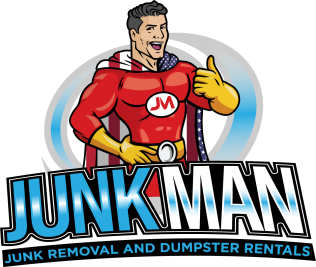The logo for a business features a muscular superhero mascot at its center, who embodies the spirit of "Junkman." He is clad in a red leotard, yellow gloves, and a yellow belt with a silver buckle. The superhero, with his dark, close-cropped hair and confident smile, flashes a thumbs-up with his left hand, while his right hand rests on his waist. Draped around his neck is a cape resembling the American flag, with its red, white, and blue colors vividly displayed. A bold "J.M." is emblazoned on his chest in red lettering on a white background. Encircling the superhero is a dynamic swirl graphic, featuring shades of gray, white, and blue, which adds a sense of motion and cohesion to the design. Below the superhero, large text reads "Junkman" in blue and white, and underneath this, in blue text on a black line, are the words "junk removal and dumpster rentals." The overall design reflects both a sense of strength and patriotic pride, set against a primarily white backdrop.